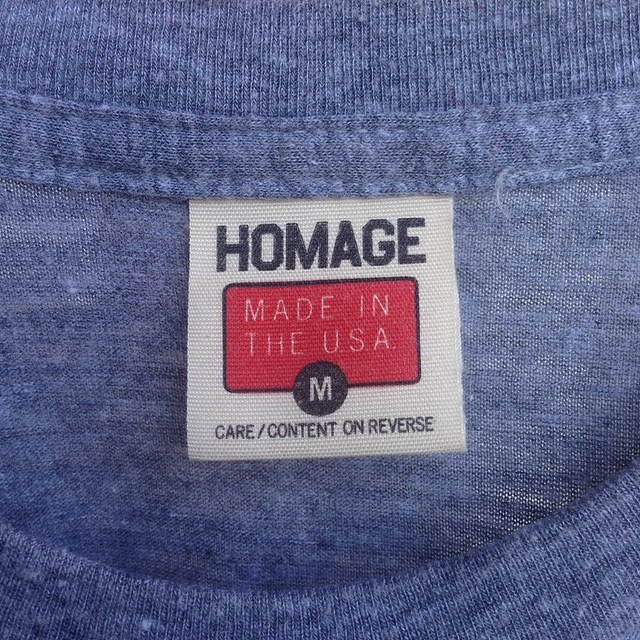The image is an indoor, close-up photograph showcasing the label inside the neck area of a medium-sized, blue cotton t-shirt. The t-shirt has a soft, light, and somewhat loosely woven fabric, reminiscent of denim, allowing light to shine through small, fine holes in some areas. The white, square label is prominently positioned at the back of the shirt's collar, which is visible and has a rounded half-circle shape. It features the brand name "HOMAGE" in large, blue capital letters at the top. Just below that is a red rectangle with a black outline, inside which "MADE IN THE USA" is written in yellow capital letters. A black circle, enclosed by this rectangle, contains a white capital "M" indicating the medium size. Beneath this, the label reads "CARE/CONTENT ON REVERSE" in black letters. The shirt appears brand new and is depicted in sharp focus.